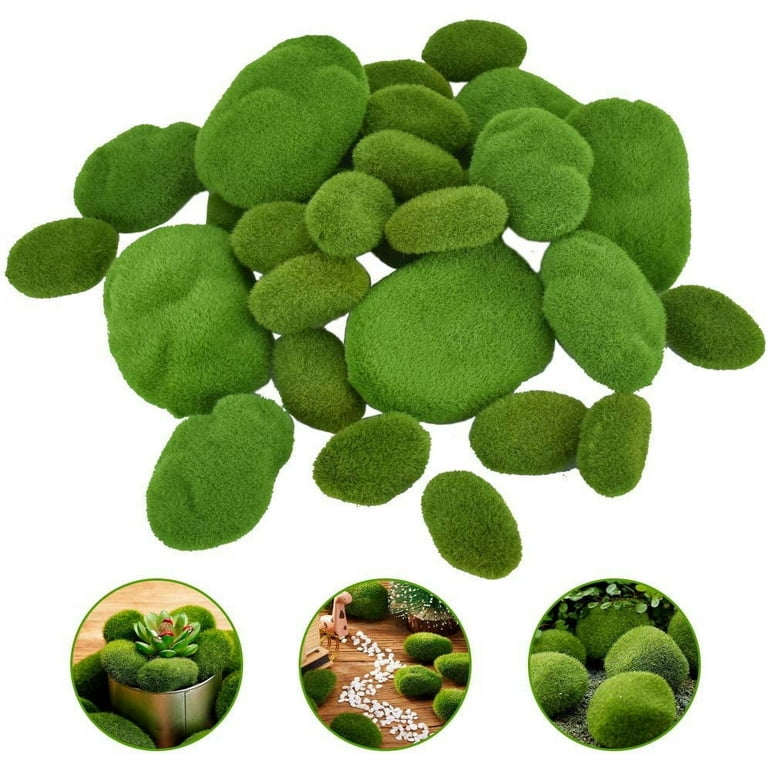The image depicts a collection of green, felt-covered rocks resembling pebbles or mossy stones. These artificial rocks vary in size, with some small and oval-shaped, and others larger and more rounded. The top portion of the image features approximately 20 to 30 of these rocks arranged over a white background. Below this main image, there are three smaller circular insets bordered in green, each showcasing various uses for these decorative items. 

The first circle on the left displays a silver container filled with smaller green felt rocks arranged like flower petals, with a succulent plant placed in the center. The second, central circle shows green felt rocks alongside white rose petals on a wooded surface, creating a decorated area. The third circle on the right features a garden scene where these green rocks are scattered among foliage and one appears to be used as a planter with leaves growing out of it. The overall composition suggests these green felt rocks can be used creatively for home and garden decoration.